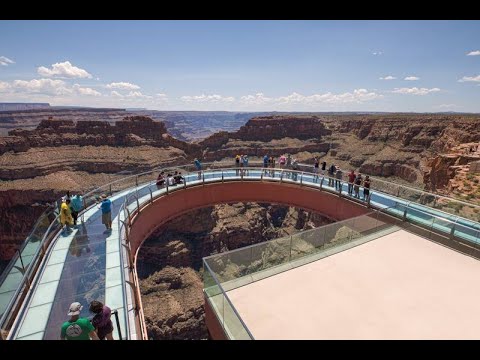The image portrays a breathtaking scene at the Grand Canyon, showcasing the iconic U-shaped glass skywalk. The skywalk extends over the canyon, providing a dramatic view straight down through its transparent floor. Numerous tourists, clad in colorful casual attire and hats, are scattered along the bridge, peering through the glass at the awe-inspiring canyon below. The backdrop features the expansive Grand Canyon with its striking southwestern palette of burnt sienna and purples, set against a clear blue afternoon sky dotted with distant, low-hanging white clouds. To the right of the skywalk, a light tan-colored platform with a glass railing offers a more solid viewing experience for those who prefer not to venture onto the glass walkway. The tourists are engrossed in their experience of the natural wonder, the glass-bottom bridge making them feel as if they are floating above the canyon's majestic depths.